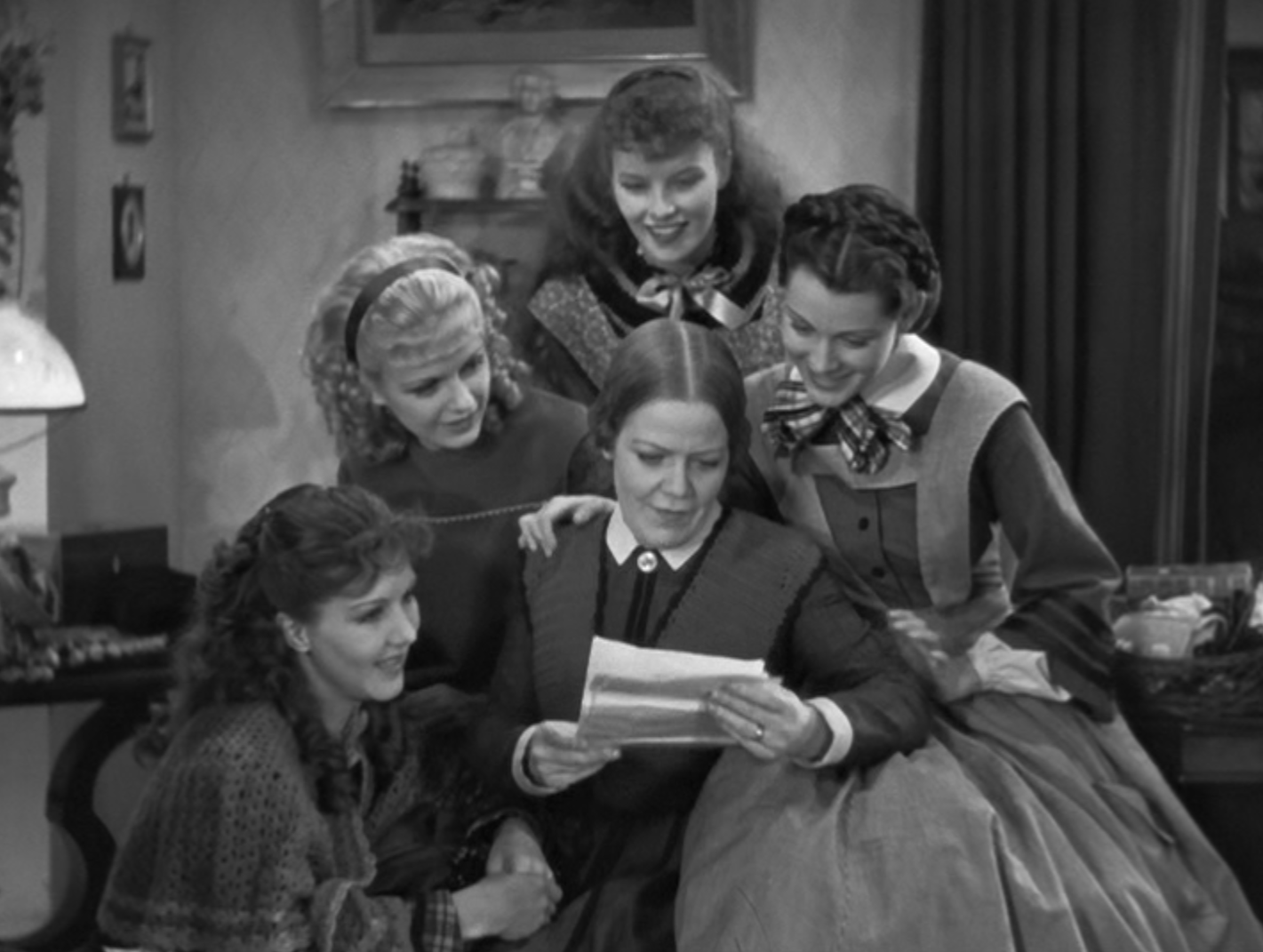This black-and-white image, possibly a still from an older movie or television show, captures a quintessential domestic scene set in what appears to be the 1930s or earlier. The central figure is an older woman, potentially a mother, distinguished by her wedding ring, who is seated and engrossed in reading a letter. Surrounding her are four younger women, bearing cheerful and curious expressions as they peer over her shoulder to catch a glimpse of the letter. 

The women are all adorned in period-appropriate clothing and hairstyles that evoke a bygone era. The living room setting is meticulously detailed with vintage furnishings: an old-fashioned lamp on a table, long dark curtains likely covering a window, picture frames of various sizes adorning the walls, and shelves filled with statues and other home décor items. This vividly nostalgic tableau offers a snapshot of familial bonds as they gather in their timeless living room, immersed in a shared moment of intrigue and warmth.